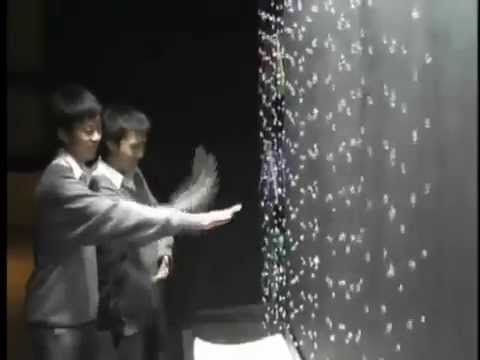The image, taken in a dark room that resembles a museum, features two young Asian men, possibly of Taiwanese, Japanese, Chinese, or Korean descent, standing in front of a striking art installation. Both men are wearing gray shirts with white collars, suggesting school uniforms or formal attire. They have short black hair and tan complexions.

In the left-hand corner of the photo, they are depicted interacting with a captivating display—a man-made waterfall or curtain of cascading water droplets or beads, illuminated against the predominantly dark background. The water or beads fall in a vertical line on the right side of the image, with individual droplets clearly visible and a basin or white object at the bottom catching the water.

Despite the low resolution and slight blur, the image captures the men smiling and waving their hands just above this luminous curtain. The lighting in the room primarily focuses on the display and the area immediately around it, leaving the rest of the space in shadow. This artistic composition, along with the men's engagement with the installation, contributes to the overall dynamic and immersive quality of the photograph.